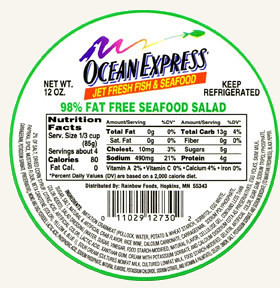This square-shaped image, viewed from an overhead perspective, prominently features a sticker with intricate details. Dominating the image is a large green circle set against an off-white background. Within this circle, a decorative rainbow squiggly line adorns the top, accompanied by a green fish that matches the circle’s color. Below this artistic touch lies the bold logo "Ocean Express," rendered in black with a purple drop shadow for emphasis.

Further down, the text "Jet Fresh Fish and Seafood" is displayed in a vibrant yellow font set against a striking red background. Additional details flank either side of the central information: "Net Weight 12 ounces" is positioned on the left, and "Keep Refrigerated" is on the right. Just beneath the main logo, the phrase "98% Fat-Free Seafood Salad" is highlighted in green.

The center of the sticker features a rectangular box containing the nutrition facts, while the bottom half is densely packed with a spiraling list of ingredients, forming a semicircular pattern. The sticker likely adorns the top of a container, rich with information and eye-catching design elements.